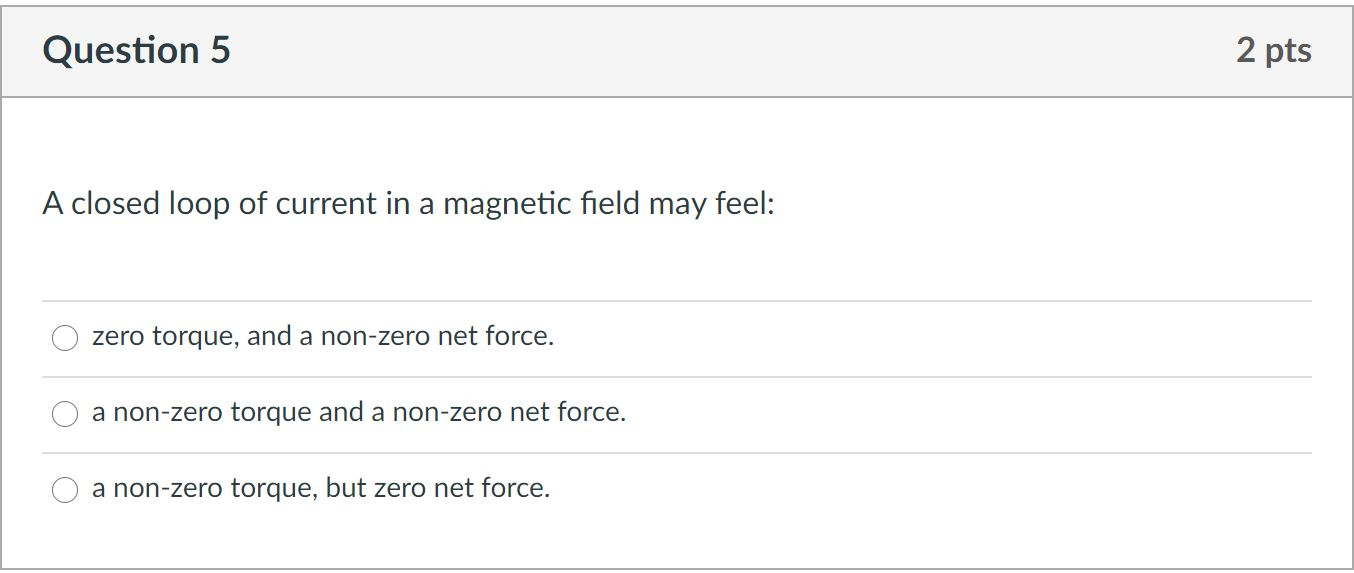The image displays what appears to be a school quiz question formatted within a rectangular box. The box has a gray header at the top, where "Question 5" is labeled in black on the left-hand side. On the far right-hand side of the header, "2 PTS" (indicating two points) is written. 

Below this header, the rest of the box is white with black text. The question presented reads: "A closed loop of current in a magnetic field may feel:" followed by a colon. Three multiple-choice options are provided, each marked by an empty circle for selection, and separated by lines.

The first option reads: "Zero torque, and a non-zero net force."
The second option reads: "A non-zero torque and a non-zero net force."
The third option reads: "A non-zero torque, but zero net force."

At this point, none of the options have been selected yet. The entire quiz question is presented in a consistent font style, with variations only in text size and highlighting.